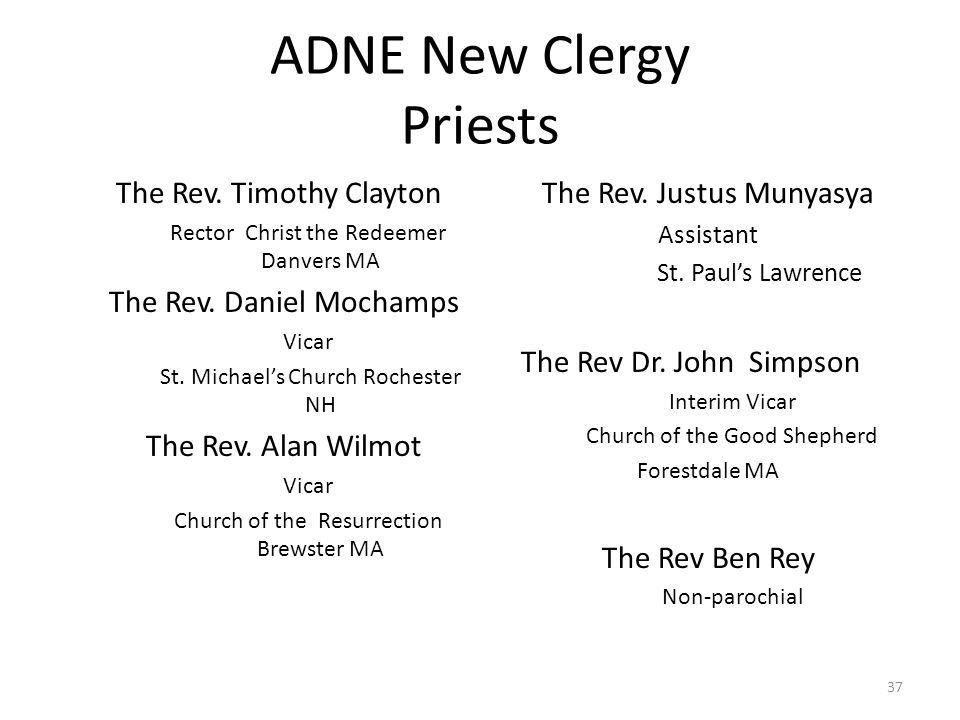The image is a church-related listing, designed as a text-based announcement on a white background. The text, presented in uniform black font varying only in size for emphasis, is headed by "ADNE New Clergy Priests" in bold, capital letters. Beneath this title, the names and titles of six clergy members are organized into two columns, each listing three names. 

The left column includes:
1. The Reverend Timothy Clayton, Rector, Christ the Redeemer, Danvers, MA.
2. The Reverend Daniel Mochamps, Vicar, St. Michael's Church, Rochester, NH.
3. The Reverend Alan Wilmot, Vicar, Church of the Resurrection, Brewster, MA.

The right column includes:
1. The Reverend Justice Muniasa, Assistant, St. Paul's, Lawrence.
2. The Reverend Dr. John Simpson, Interim Vicar, Church of the Good Shepherd, Forestdale, MA.
3. The Reverend Ben Ray, Non-Parochial.

Each clergyman's name is followed by their respective title and the church or parish they are associated with, providing a clear and organized listing of new clergy priests within the ADNE.